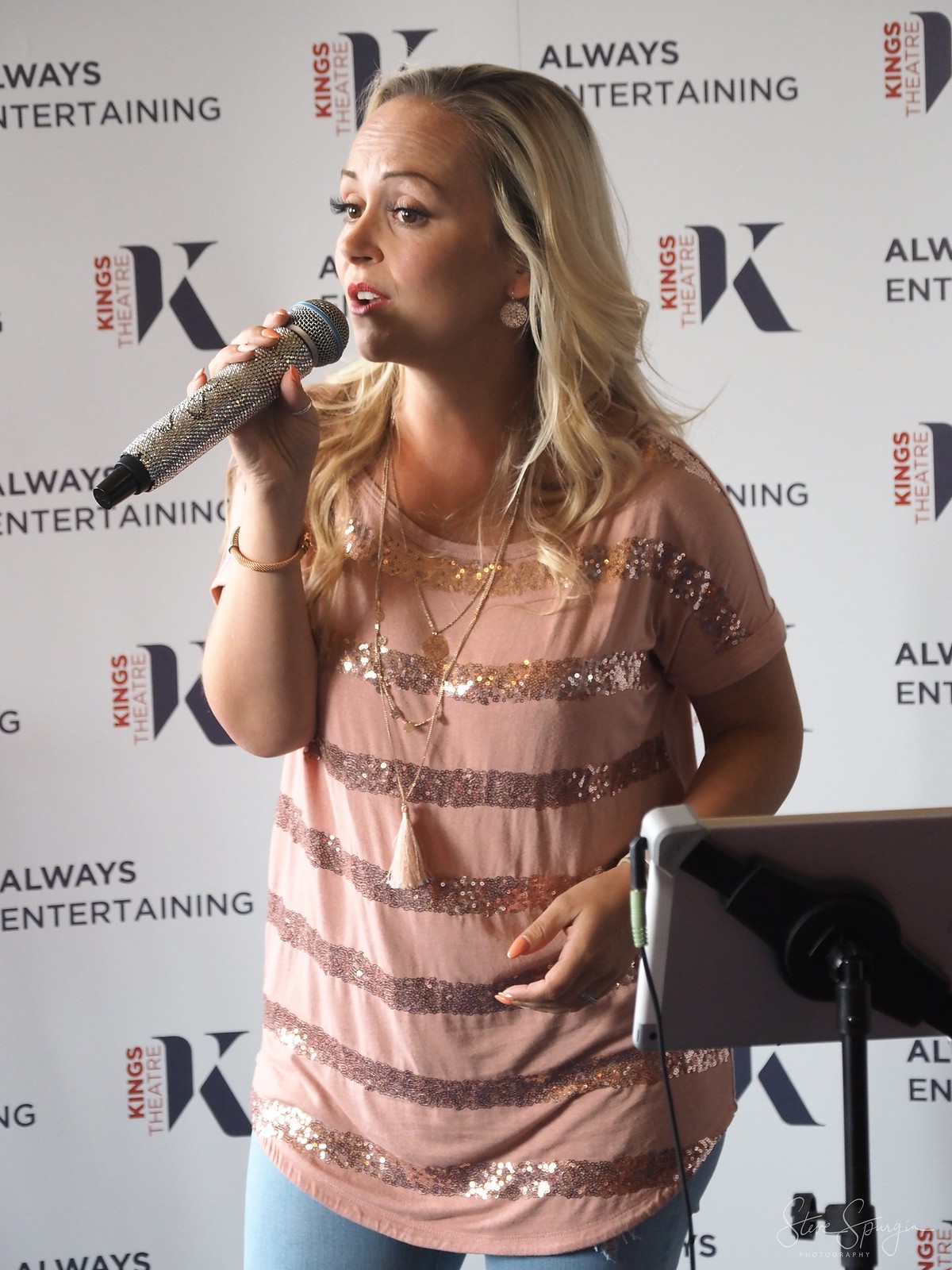In this vertical rectangular image, a young blonde woman is captured mid-performance in what appears to be a recording studio or tryouts for King's Theater. She has long blonde hair with darker roots that reaches to about the top of her chest. Her eyes sparkle with enthusiasm as she holds a silver microphone close to her lips, its black base contrasting against the metallic sheen. She is adorned in a vibrant, pink top with gold, glittery horizontal stripes, paired with jeans, and her nails are painted a soft, peach color. On her wrist, she wears a bracelet that adds a touch of elegance to her outfit. Behind her, the backdrop features a white wall with the King's Theater logo and the tagline "Always Entertaining" in bold letters. To her side, stands a mechanical apparatus supporting what appears to be an iPad, possibly displaying lyrics for her performance. Despite the tech assist, she exudes confidence as if she knows the song by heart, making it seem like a joyous audition for a musical. The atmosphere is filled with excitement and anticipation, highlighting a moment of passion and artistry.